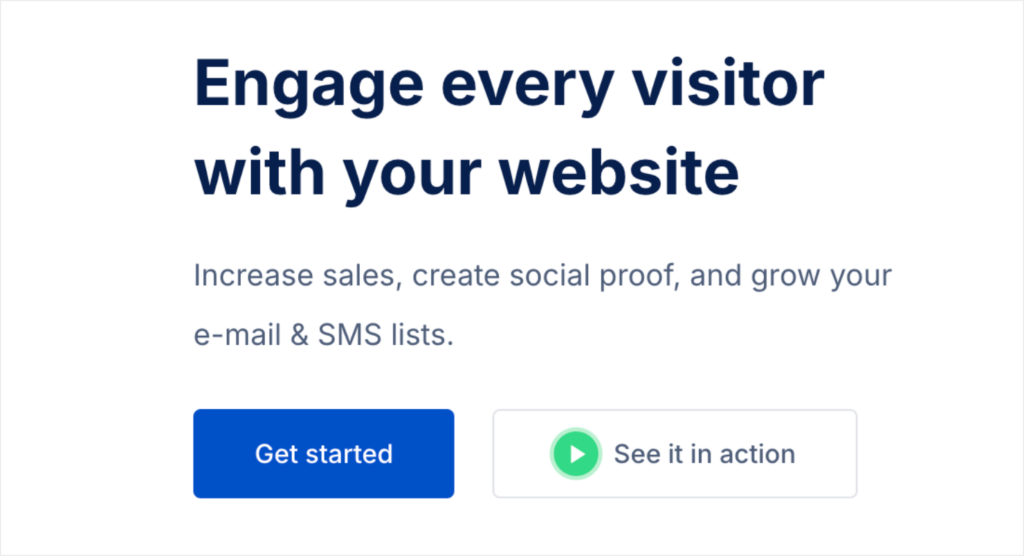The image contains a minimalistic, clean white background with a central message designed to captivate viewers. At the top, a two-line headline is prominently displayed in large, bold, blackish-blue text that reads: 
"Engage Every Visitor with Your Website."

Beneath this primary headline, a concise, grey subheading provides additional information over two lines:
"Increase sales, create social proof, and grow your email and SMS lists." 

Below this subheading, two interactive buttons are presented. On the left, there's a smaller, blue button with "Get Started" written in white text. Adjacent to it, on the right, there's a white button outlined by a thin grey border. This button features a play icon—a white triangle pointing to the right encircled by green—and to its right, the grey text "See it in Action."